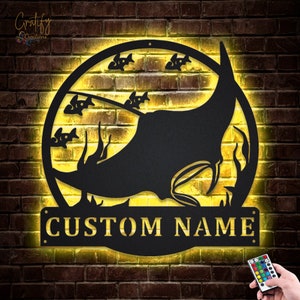The image depicts a circular ironwork wall sculpture designed as a custom piece of art. Centered within the dark iron frame is a detailed depiction of a stingray, accompanied by small baby fish. Below the stingray, the frame features a customizable text area labeled "custom name." The sculpture is mounted on a dark red brick wall, and it appears to be backlit with a yellow, fire-like illumination. In the top left corner, there's a cursive signature written in yellow. In the bottom right corner, a right hand holds a white remote control with several RGB color buttons, suggesting the lighting behind the sculpture is controllable. The entire scene suggests this is an advertisement for customizable, illuminated metal frame artwork.